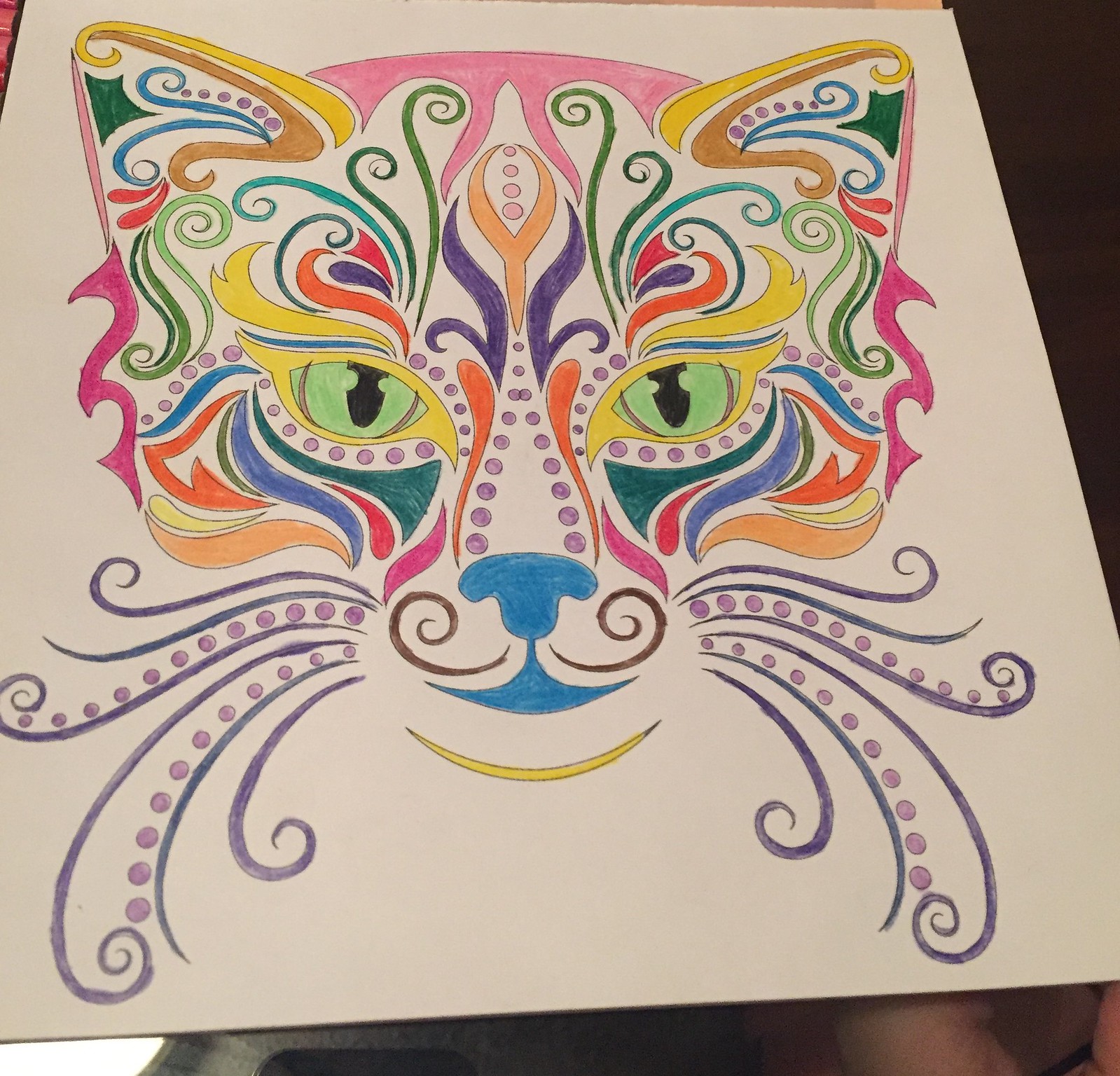The image captures a highly detailed and colorful drawing, likely created with colored pencils, depicting the head of a cat or possibly a tiger. The artwork sits on a white piece of paper, which is held by a person with a light skin tone, against a dark gray, flat-surfaced background, possibly a table. The drawing is rich in vibrant hues: the ears feature a yellow border, with brown, blue, purple, green, and orange insides. Central to the image is the animal's head, which is predominantly pink on top. Its eyes are green, surrounded by a yellow eyebrow area, and further accentuated by purple dots extending around the eyes and down the face. The whiskers, drawn with purple lines and dotted accents, frame a blue nose and blue mouth. Additionally, a brownish handlebar mustache-like pattern adorns the snout, which is also marked by purple beads or circles. The detailed and symmetrical design showcases a multitude of colors and patterns, making the face both striking and harmonious. The image occupies the majority of the photograph, extending from the bottom right to the top left.